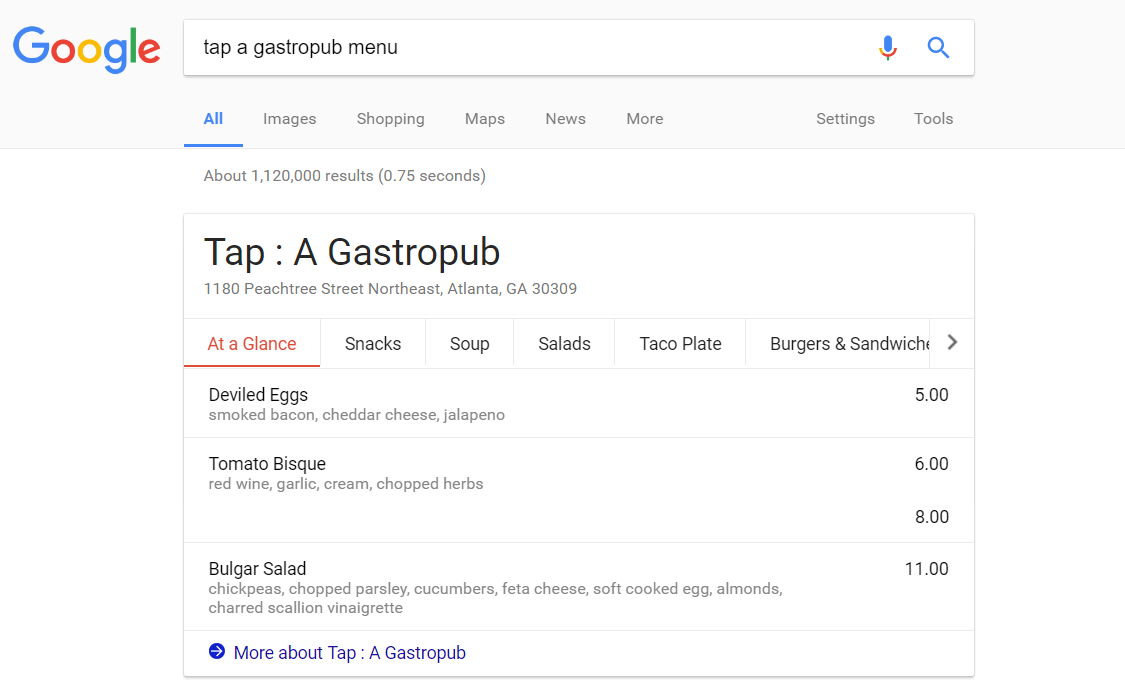In the top left corner of the image, the Google brand name "GOOGLE" is prominently displayed. Below it, a search bar contains the phrase "gastropub menu" with icons for a microphone and a magnifying glass beside it. The word "All" appears underlined in blue, indicating the current search category. Next to it are the options: Images, Shopping, Maps, News, More, Settings, and Tools.

The search results indicate approximately 1,120,000 results found in 0.75 seconds. The text "tap, two circles after that, two tiny dots, a gastropub" appears, followed by the detailed location "1180 Peachtree Street, Northeast Atlanta, Georgia, 30309."

Under the header "At a Glance," highlighted in red and underlined, different sections of the menu are listed: Snacks, Soup, Salads, Taco Plate, Burgers, and Sandwiches.

For the snacks section:
- Deviled Eggs: Smoked bacon, cheddar cheese, jalapeño, priced at $5.

For the soups:
- Tomato Bisque: Described with red wine, garlic, cream, and chopped herbs, priced at $6.

For the salads:
- Bulgar Salad: Includes chickpeas, chopped parsley, cucumbers, feta cheese, a soft-cooked egg, almonds, and charred scallion vinaigrette, priced at $11.